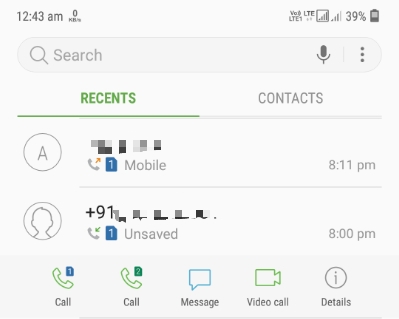This image is a detailed screenshot from a website interface, likely depicting a mobile communication app. The upper portion of the screenshot features a consistent light gray background. At the top left, the timestamp reads "12:43 AM," accompanied by a network speed indicator showing "0 KB/s" (with "KB" capitalized and "s" in lowercase). On the top right, various status icons are displayed, including "VO LTE1" and "LTE" indicators, a cell signal icon, and a battery status of "39%."

Below this status bar is a search area. It features a search bar labeled with a magnifying glass icon and the word "Search," followed by a microphone icon and three vertical dots representing additional options. 

Continuing downwards, there is a navigation menu with two tabs: "RECENTS," highlighted in green text with a green underline, and "CONTACTS," displayed in gray.

The main content area includes user-specific details. It starts with an outlined circle containing the letter "A," and a pixelized username. Underneath this, a yellow upward arrow icon is shown next to a telephone symbol and a SIM card icon labeled "1 Mobile," with the time "8:11 PM" beside it. Another circular icon below this features a person’s silhouette, with a pixelized phone number starting with "+91." Adjacent to this, a green downward arrow icon is shown with a phone and a SIM card labeled "Unsaved," and the time "8:00 PM" next to it.

At the bottom of the screenshot, there are action buttons labeled "Call," "Message," "Video Call," and "Details."